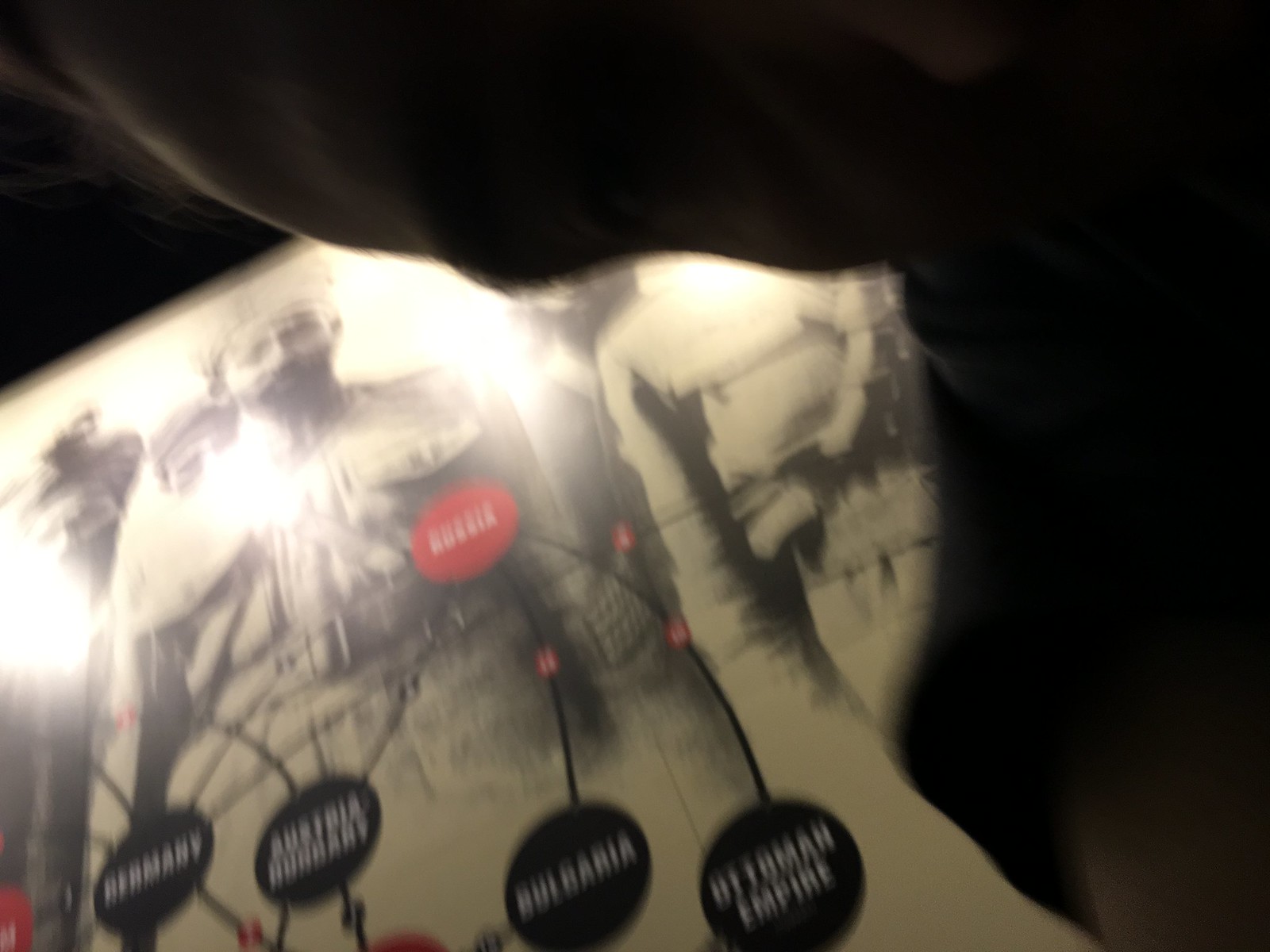The image depicts an old, sepia-toned photograph that seems to be from a historical military context, possibly World War II. The primary focus is on several soldiers in uniform, with visible details such as big pockets and mustaches. The soldiers' faces and part of their torsos are discernibly seen, though one face is partly obscured by a dark piece of fabric, possibly an arm, draped diagonally over the right corner of the photograph. The bottom part of the photo is slightly out of focus, adding to the aged appearance.

Superimposed on the image are a series of red and blue circular labels connected by dark lines, representing different countries. The most prominent circle is red with white text labeled "Russia." Surrounding it are blue circles with white text, each linked back to the Russia circle. These include "Germany," "Austria-Hungary," "Bulgaria," and "Ottoman Empire." The intricate network of circles connected by lines suggests a map-like depiction of alliances or connections between these nations during the war. The photograph appears to be held at an angle on a black surface, contributing to its dynamic composition.